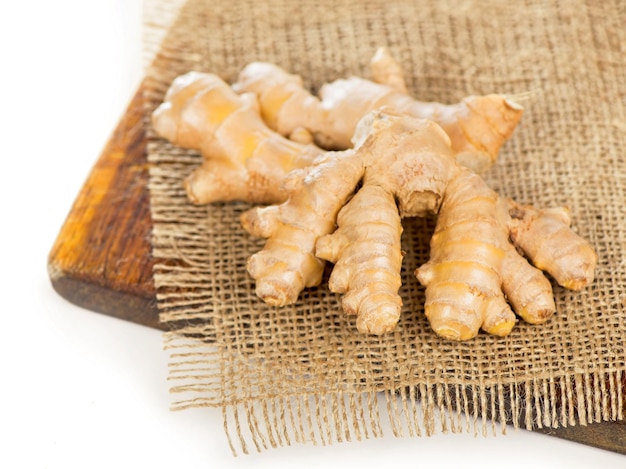The photograph captures a detailed and close-up view of a light brown, irregularly shaped ginger root with bulbous, knobby protrusions and a rugged surface texture. The ginger root rests on a burlap-like cloth, characterized by its coarse and interwoven texture. This fabric is placed atop a dark wooden board, possibly a cutting board or tabletop, providing a rustic setting that highlights the natural, earthy appearance of the root. The image emphasizes the distinct features of the ginger, such as its bumpy exterior and beige color, suggesting it is ready for culinary or medicinal use.